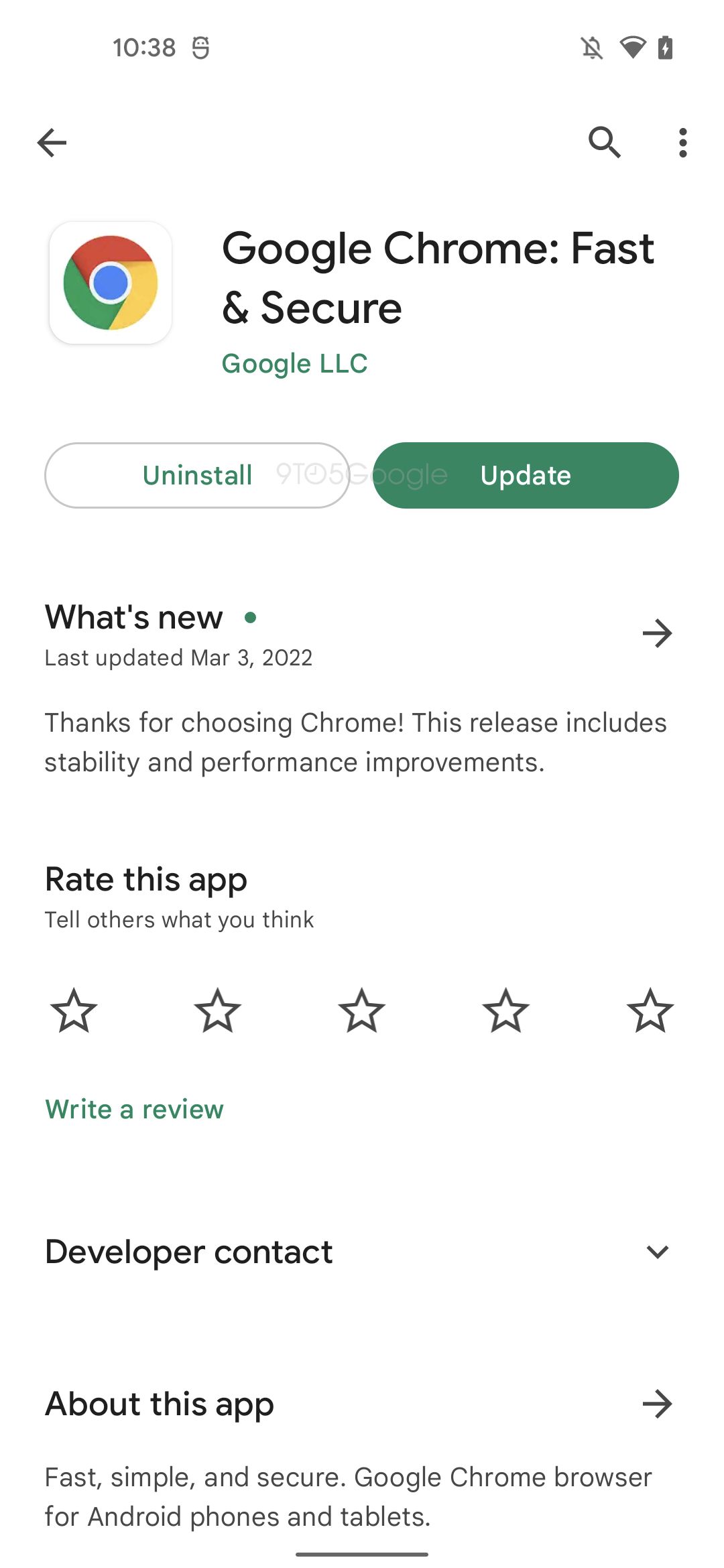The time displayed in the upper left center of the screen is 10:38. The battery icon is nearly depleted but is currently charging, indicated by a lightning bolt symbol in the center of the icon. To the left is a back arrow, followed by the Google Chrome logo, which features a red, yellow, and green circle encompassing a smaller blue circle in the center.

On the right side of the screen, there is the text "Google Chrome: Fast & Secure." Directly beneath this, "Google LLC" is displayed in green text. Below that, there are two buttons: one labeled "Uninstall" in a horizontal oval, and another green oval labeled "Update" in white text. 

Further down, the caption reads, "What's new?" accompanied by a small green asterisk. It notes that the last update was on March 3rd, 2022, and includes a message thanking users for choosing Chrome. This release contains stability and performance improvements.

The section "Rate this app" features five stars below it and a green text link labeled "Write a review." There is also an expandable section titled "Developer contact," indicated by a downward arrow, followed by "About this app." The description reads, "Fast, simple, and secure Google Chrome browser for Android phones and tablets," with the word "tablets" underlined for emphasis.